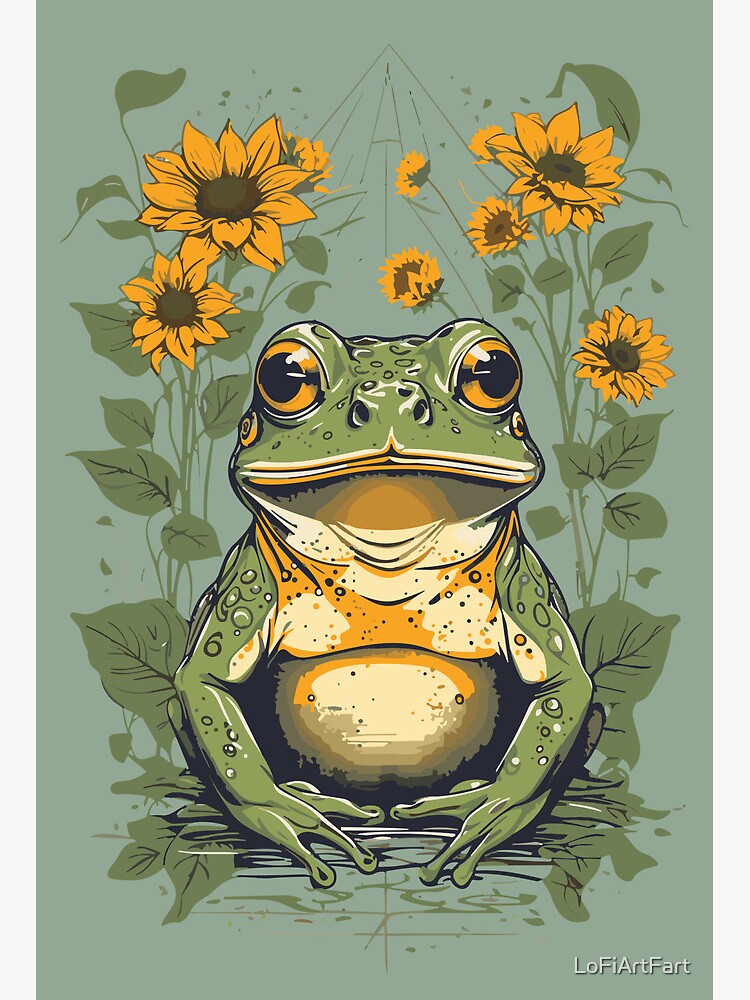In this charming outdoor scene rendered in a detailed, cartoon-like drawing, a happy green frog takes center stage, sitting contentedly in a bit of water that ripples around him. The frog, facing directly at the viewer, has black eyebrows and striking orange irises. His wide-open mouth suggests a joyful demeanor. His belly and breast display a mix of yellow, orange, and white hues, with additional white spots scattered across his green body. Surrounding the frog is a vivid array of sunflowers, with two on the left and five on the right, each adorned with yellow-orange petals and a black center. Green leaves and plants complement the bright flowers. The background is a soothing blend of greenish-blue, enhancing the lively outdoor ambiance. In the bottom right-hand corner of the image, the text reads "Lofia Artfat."